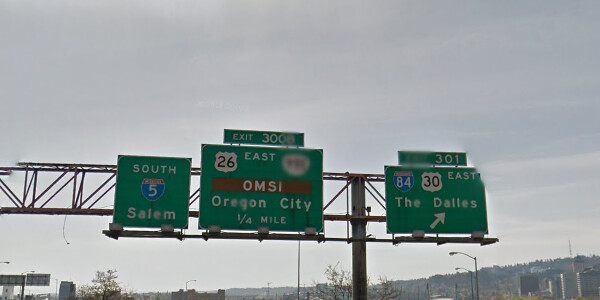The photograph showcases a section of an interstate, framed by several green traffic signs overhead. In the distance, mountains with scattered buildings rise under a heavily overcast sky, which appears almost completely white. In the lower left-hand corner, a few indistinct billboards can be seen in the background. Three prominent green traffic signs dominate the foreground: the left sign directs drivers to "South 5 Salem," the middle sign announces "Exit 326 East OMSI Oregon City, 1/4 mile," and the right most sign indicates "Exit 301, 8430 East, The Dalles" with an arrow for guidance.